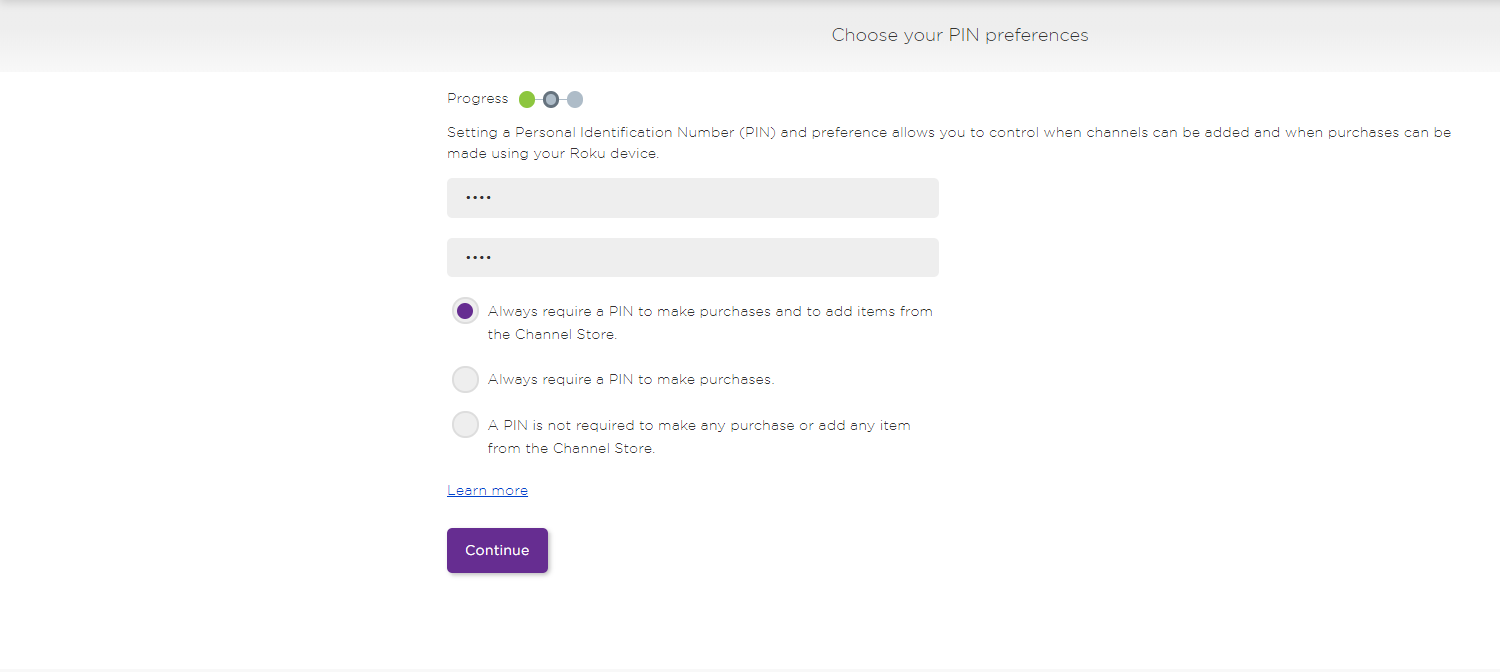This image is a screenshot taken from a user's computer, displaying the top section of a Roku device settings page titled "Choose Your PIN Preferences." The acronym "PIN" is prominently displayed in uppercase letters. The interface features a visual progress tracker, with three dots indicating different stages. The current stage is highlighted with a green dot, while the subsequent stages are marked by an unfilled blackish-purple dot and a gray dot, respectively.

Below this, a detailed explanation reads: "Setting a Personal Identification Number (PIN) preference allows you to control when channels can be added and when purchases can be made using your Roku device." This is followed by two input boxes, each containing four placeholder dots, presumably for entering the PIN.

Further down, the screen displays options for PIN preferences. The first option, highlighted by a filled purple dot, states "Always require a PIN to make purchases and to add items from the Channel Store." The second option, marked by an empty gray dot, reads "Always require a PIN to make purchases," but this option is not selected. The final option says "A PIN is not required to make any purchases or add any items from the Channel Store."

The bottom of the screen features a "Learn more" link and a prominent purple "Continue" button.